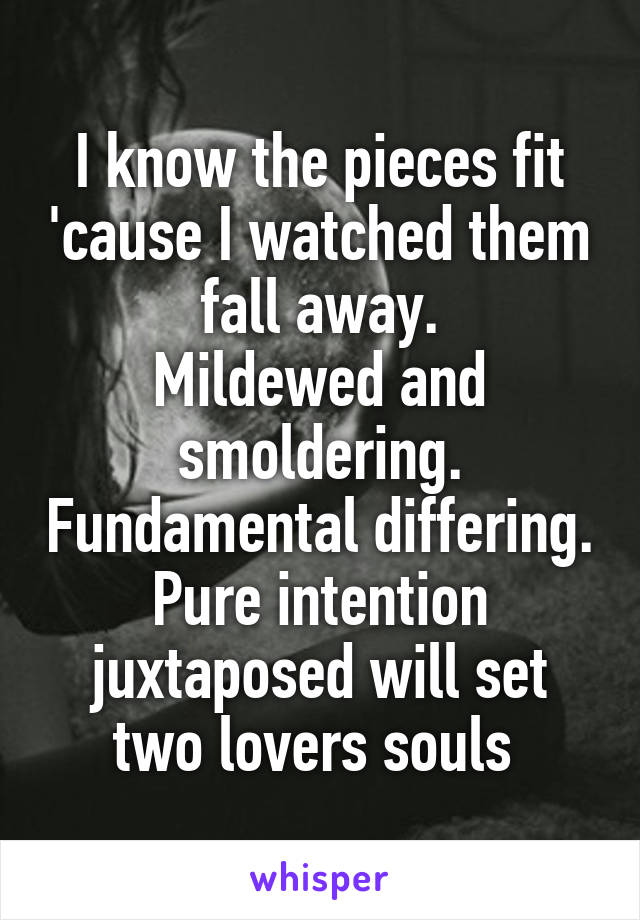The image is a black and white, heavily edited photograph depicting a woman sitting down and holding a moon roughly the size of a beach ball. Superimposed over this vague, dark background is a motivational poem, written in bold white text: "I know the pieces fit because I watched them fall away, mildewed and smoldering, fundamental differing, pure intention juxtaposed will set two lovers' souls." Below the text is a small white box featuring the word "whisper" in lowercase, purplish-blue letters.